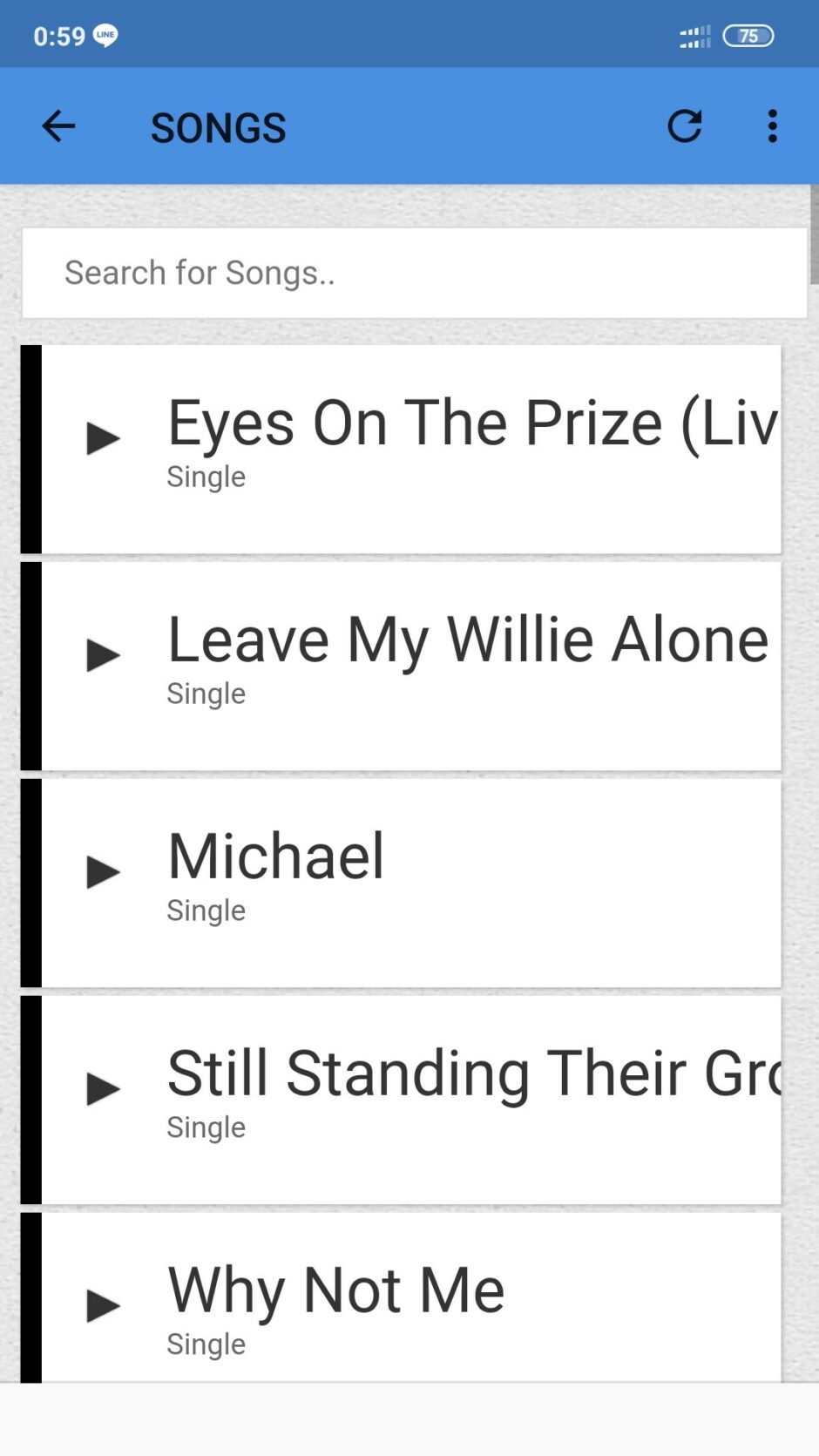The image displays a digital music interface, starting with a blue border at the top. The time, "05:59," is displayed within this border. Below the time, the interface has a light blue area featuring a left-pointing arrow labeled "Songs." Nearby, there is a refresh button, and in the upper right corner, there is a vertical ellipsis (three dots).

The main section of the interface has a gray background with a search bar, inviting the user to "Search for songs." Beneath the search bar, there are five rectangular areas, each representing a different song. These rectangles are white with a black strip running vertically along the left side. To the right of each black strip, there is a play button, followed by the song title in bold black text. Below each song title, the word "Single" appears in gray text.

The song titles listed from top to bottom are:
1. "Eyes on the Prize (Live)"
2. "Leave My Willy Alone"
3. "Michael"
4. "Still Standing" (with the rest of the title cropped out and ending with "Gr")
5. "Why Not Me"